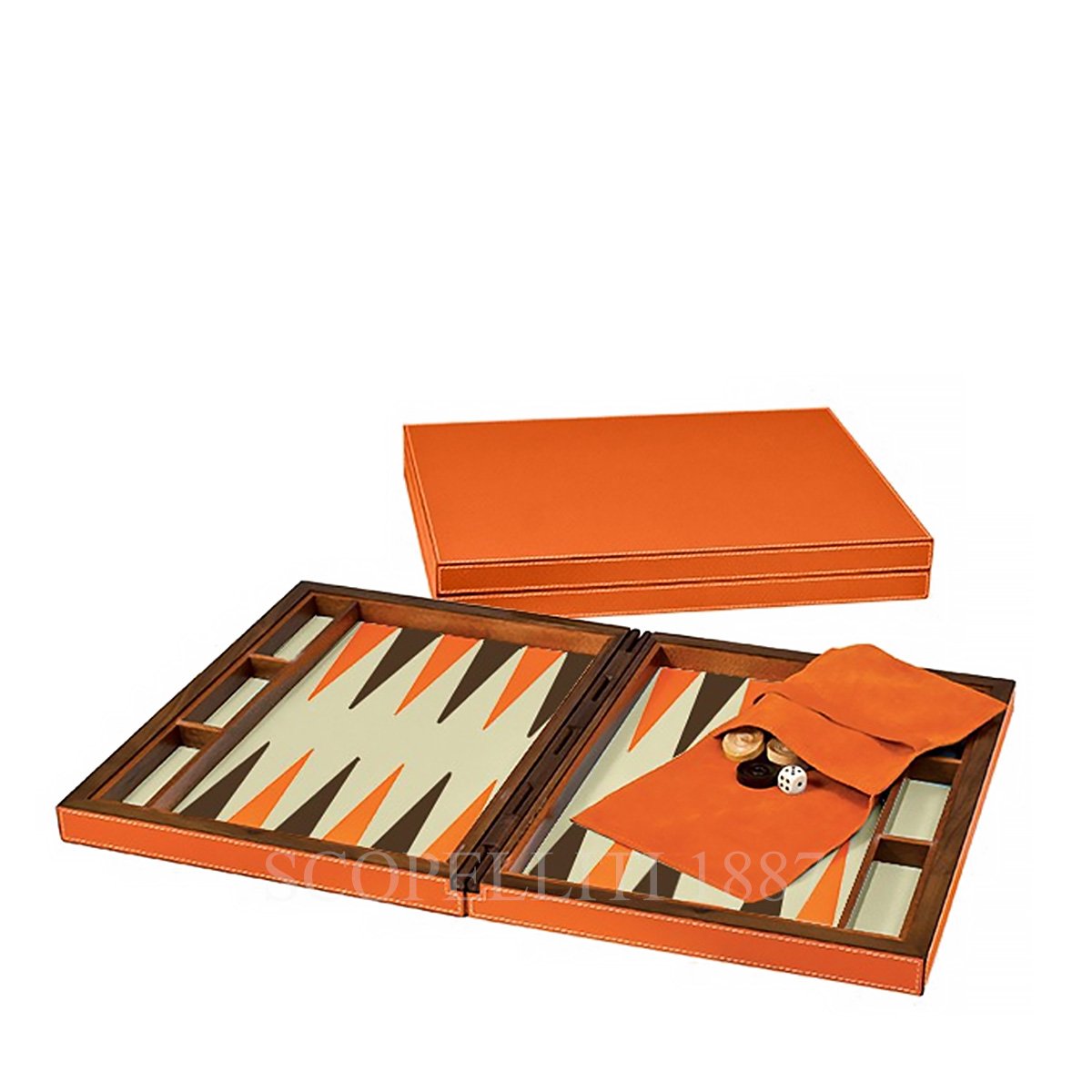The image depicts a backgammon set on a white background. The set includes an orange case that is shown both closed and open. When open, the interior reveals a game board with a wooden base featuring distinctive orange and white patterns, along with black and orange triangles where the pieces are placed. The board is designed with three small trays on either side for each player. Inside, there is an orange pouch used to store the black and tan playing pieces and dice. Despite mentions of the case typically having a latch, it is not visible in the image. Additionally, a semi-transparent watermark with the text "Scopeletti 1887" is faintly visible overlaying the picture. The image also includes what may be a red box or bag, suggesting either packaging for or as components of the backgammon game.